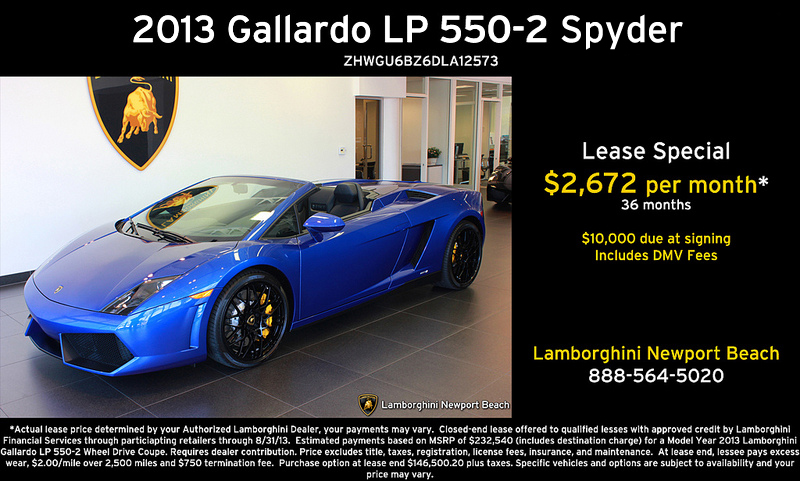This is an advertisement for a 2013 Royal Blue Lamborghini Gallardo LP 550-2 Spyder, set against a black backdrop. The sleek, aerodynamically shaped two-door convertible, featuring black leather seats with the top down, is prominently displayed in a Lamborghini dealership. Across the top of the image, in white text, is the model name "2013 Gallardo LP 550-2 Spyder" followed by a serial code "ZHWGU6BZ6DLA12573". To the right of the car, in bold white print, is the text "Lease Special" with the lease price "$2,672 per month," detailed as a 36-month lease with $10,000 due at signing, which includes DMV fees, in yellow print. Below this, the dealership name "Lamborghini Newport Beach" and the phone number "888-564-5020" are listed. At the bottom of the image, fine print explains the lease terms, including specifics about the MSRP, additional fees, and conditions for qualified lessees through Lamborghini Financial Services, valid until 8-31-13. The fine print also includes information on the purchase option and possible additional charges for excess mileage and termination.